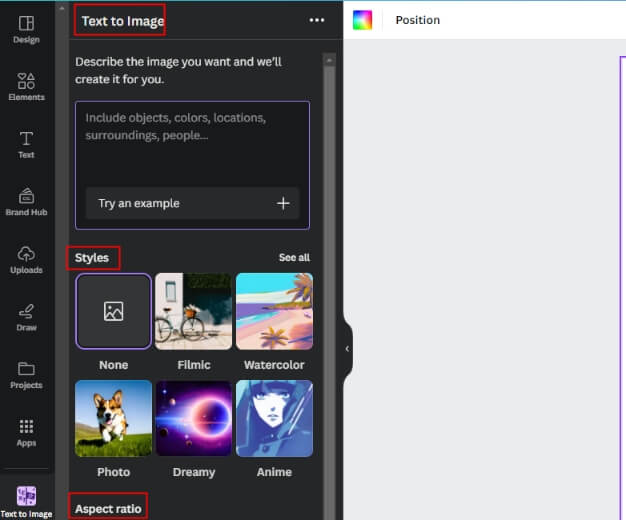The image is a screenshot of an editing application interface. At the top of the interface, a vertical toolbar is displayed on the left side of the screen with various sections labeled: Design, Elements, Text, Brand Hub, Uploads, Draw, Projects, and Apps.

The focal point of the screenshot includes a prominent red outline around the "Text" section of the toolbar. Adjacent to this section, there's a highlighted area with the text: "Describe the image you want and we'll create it for you." Beneath this prompt is a text box that instructs users to "include objects, colors, locations, surroundings, people," providing clear guidelines for curating the description.

Towards the bottom of the interface, there's another red box around the "Styles" section, which offers various creative options such as None, Filmic, Watercolor, Anime, Dreamy, and Photo. Further down, there's yet another red box highlighting "Aspect Ratio" settings.

An additional note at the lower section of the screen encourages users to "Try an example," indicated with a plus sign (+) on the right side.